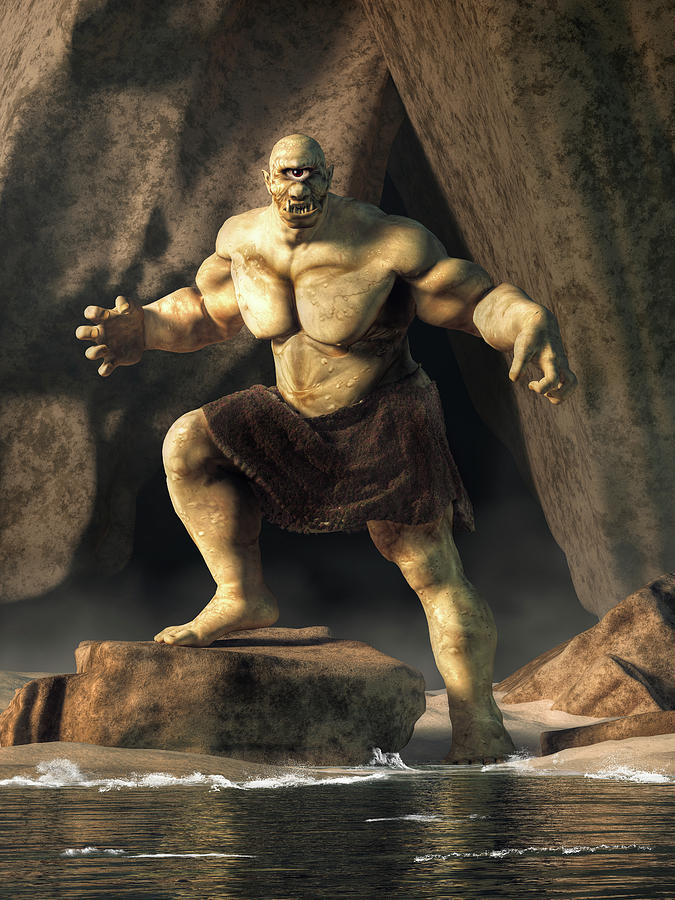This illustration depicts a terrifying Cyclops creature standing on a rock at the water's edge, right outside the entrance of a triangular cave. The Cyclops, presumably male, exudes a menacing aura with its grotesquely muscular physique. Its greenish-tan skin and lack of body hair highlight the sheer massiveness of its torso, biceps, and chest. The creature's single, glaring eye is centered on its small head, and it bears a mean expression with a mouth full of sharp, jagged fangs and an underbite that causes its large tusks to jut upward prominently.

The Cyclops is clad in a modest loincloth or kilt, which wraps around its enormous waist, leaving it barefoot. One of its feet is planted firmly on a flat shoreline rock, with the knee bent in a combative stance. Its powerful arms are poised for action—one arm outstretched with the palm facing forward and the other curled as if ready to grasp something menacingly.

The illustration employs an earthy color palette, with browns and faded tones, lending it an archaic, timeless feel. The ominous cave behind the Cyclops and the water lapping at its feet add to the sense of danger and fantastical dread surrounding this menacing giant.